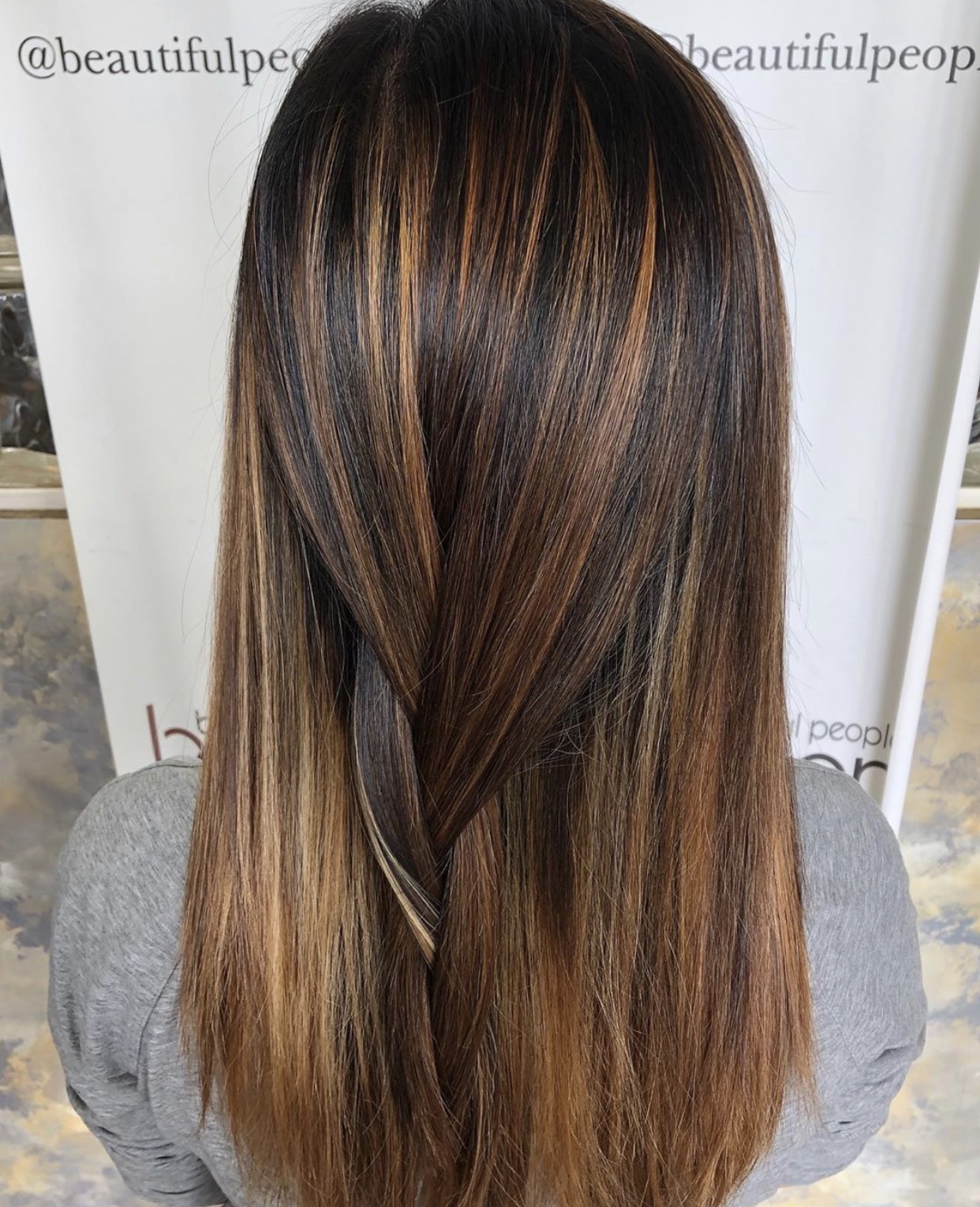The photograph features the back of a young girl seated or standing with shoulder-length, multi-colored hair that's a mix of blonde, light brown, red, and black hues. Her hair is styled in a partial braid down the back, left unfinished without a clamp, and she wears a gray shirt. The background includes a white signboard with the text "@beautifulpeople.com" written across the top. The floor beneath her is made of granite with shades of tan, brown, gray, and white, adding a sophisticated touch to the setting, possibly a salon. Some darker marble also runs around the edges of the signboard, giving the scene an enclosed appearance.